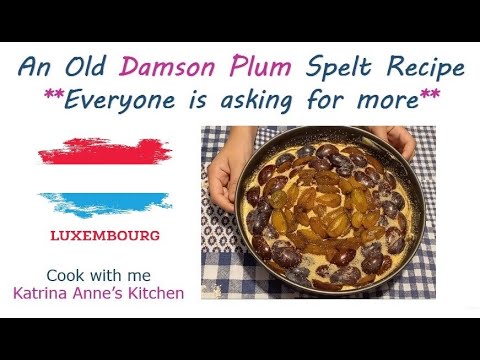This advertisement features a charming culinary scene highlighting "An Old Damson Plum Spelt Recipe." The title is visually striking with "Damson Plum" written in vibrant purple, while the rest of the text is in blue. Below the title is a line of blue text encased in asterisks proclaiming, "Everyone is asking for more."

The left side of the advertisement prominently displays a paint streak symbolizing the flag of Luxembourg, with red at the top, white in the middle, and blue at the bottom. Underneath this streak, "Luxembourg" is announced in bold, red capital letters followed by the invitation to "Cook With Me" and the name "Katrina Ann's Kitchen," both in blue and purple text that mirror the colors at the top of the image.

Central to the lower right of the advertisement is a photograph showcasing a mouth-watering dish, likely featuring the seasonal plums mentioned earlier. The dish, a black pan cradled by two hands, rests on a blue and white striped tablecloth. The edible creation, possibly adorned with sliced plums, stands atop a napkin with a white background and black circles.

The entirety of the image is neatly framed with a black band at the top and bottom, drawing focus to the culinary masterpiece and the invitation to enjoy a beloved, time-honored recipe from Katrina Ann's kitchen.